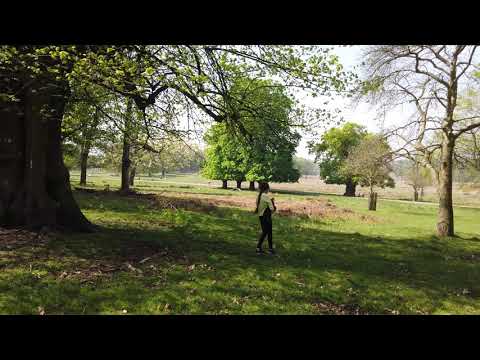In the photograph taken outdoors, a young girl with long hair, either in a ponytail or braid, walks away from the camera in a grassy park area. She wears a light lime green shirt that almost blends into the green grass around her, paired with black leggings. The girl is positioned centrally, facing away, moving towards the right side of the image. To her immediate left stands a very large, thick tree trunk, while on her right, a thinner tree without many leaves is visible. The grassy area is somewhat patchy and scattered with dead leaves and twigs. In the background, more fields with a few scattered trees can be seen under a clear sky. The scene appears to be captured in late spring or early summer, evident by the lush, dense, and healthy green leaves on several trees, contrasting with a few trees that have sparse foliage. The overall atmosphere suggests a somewhat cultivated and managed estate, indicated by the presence of very tall lime trees near what looks like a roadway running parallel to the horizon. The image is framed with large black bars at the top and bottom.